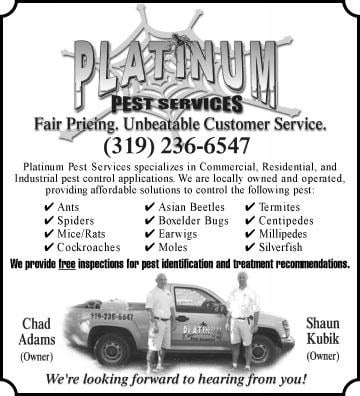This black and white advertisement for Platinum Pest Services, likely scanned from an old magazine, features a company logo at the top, where the dot on the "i" in "Platinum" is creatively replaced with a spider. Below the logo, the advertisement highlights "Fair Pricing, Unbeatable Customer Service" and provides a contact number, 319-236-6547. Platinum Pest Services, a locally owned and operated company, specializes in commercial, residential, and industrial pest control applications. They offer affordable solutions to manage a range of pests listed with check marks, including termites, silverfish, moles, cockroaches, ants, spiders, and more. The advertisement also mentions offering free inspections for pest identification and treatment recommendations. At the bottom, there's a black and white photograph of two men, Chad Adams and Sean Kubik, both owners, standing in front of a truck adorned with the company logo, symbolizing their commitment and hands-on approach to their business.